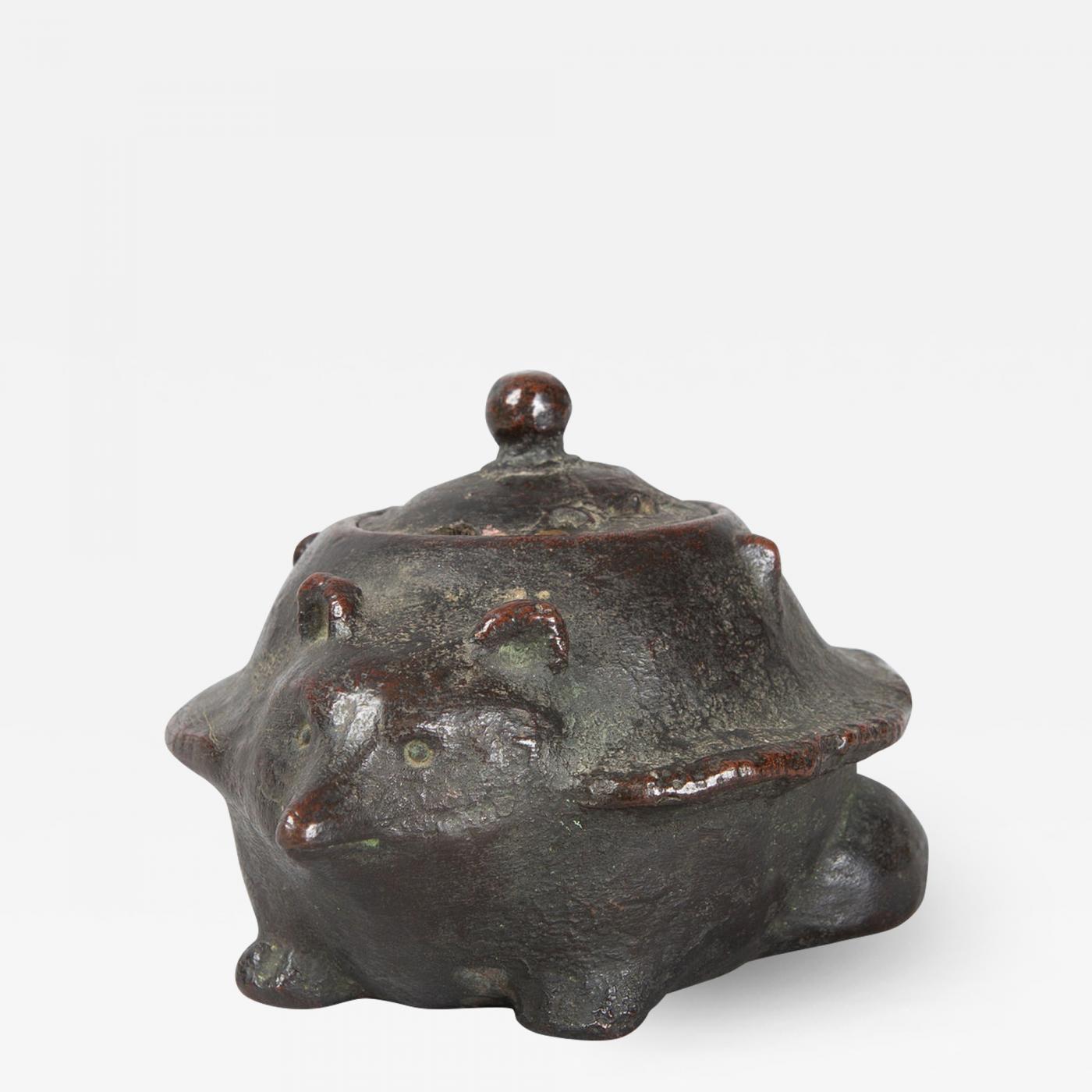The image showcases an antique, stoneware-style pot modeled after an animal, prominently set against a white background. The pot has a dark brown to black hue, indicating significant age and wear, with glimpses of a bronze-like sheen on certain areas. The pot takes on a roundish, squat shape, resembling a heavy, crude pottery item. It features a distinct lid at the top with a round knob that is slightly browner and shinier than the rest of the pot. Below the lid, we observe an animal face characterized by rounded ears, prominent yellow eyes with black pupils, and a pointed snout with a simple line for a mouth. Extending from the front are tiny feet or paws, hinting at the creature's base. The design suggests a mythical animal, potentially a mixture between a hedgehog, weasel, or badger, and is adorned with small, worn spike-like protrusions reminiscent of a turtle shell. The pot also has what appears to be a tail coiled around its back, further adding to its mythical appearance. The uneven, unglazed finish with visible wear adds to its rustic and ancient charm.